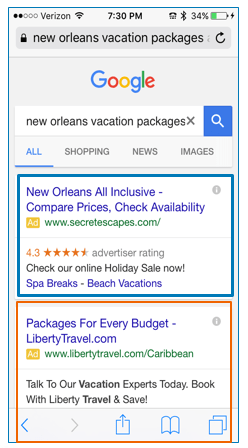This screenshot from a cell phone captures a Google search for "New Orleans Vacation Packages". At the top, the device's status bar shows five small circles—two solid black and three outlined in black—alongside the Verizon signal indicator, indicating full Wi-Fi connection. The time displayed is 7:30 PM. Additional icons include Bluetooth, a battery icon at 34% with a green background and a black lightning bolt indicating charging status, and a lock symbol.

Below the status bar, the Google search interface displays the query "New Orleans Vacation Packages" in the search bar. To the right of the search bar, there is an "X" to clear the search and a blue square with a white magnifying glass for initiating the search. The "All" tab is highlighted and underlined in blue, while the "Shopping," "News," and "Images" tabs are shown in gray.

The first search result is an advertisement outlined in a blue rectangle, promoting "New Orleans All-Inclusive Compare Prices, Check Availability" from Secret Escapes (www.secretescapes.com), accompanied by four orange stars indicating the advertiser rating. The ad mentions "Check out our holiday sale now, spa breaks, beach vacation" in yellow text.

Another ad in an orange rectangle promotes "Packages for Every Budget, Liberty Travel" with the URL libertytravel.com/caribbean in green. The ad encourages users to "Talk to our vacation experts today, book with Liberty Travel, and save."